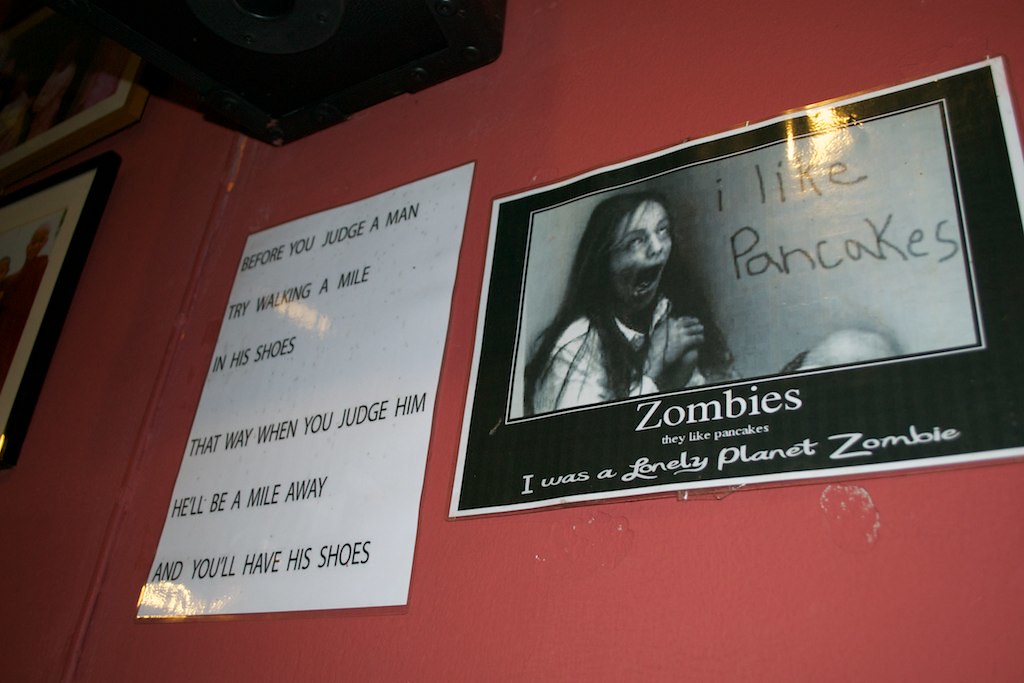This indoor photograph captures a series of posters attached to a pink wall. The poster on the left is white with black, typed text that humorously reads, "Before you judge a man, try walking a mile in his shoes. That way when you judge him, he'll be a mile away and you'll have his shoes." To the right is a laminated black-and-white poster depicting a female zombie with exaggerated and grotesque features—open mouth, funky eyes, and scars with blood. Handwritten next to her are the words, "I like pancakes." Beneath this image, the text reads, "Zombies, they like pancakes. I was a Lonely Planet zombie." Additional posters or paintings are visible further left but are partially cut off and indistinguishable.